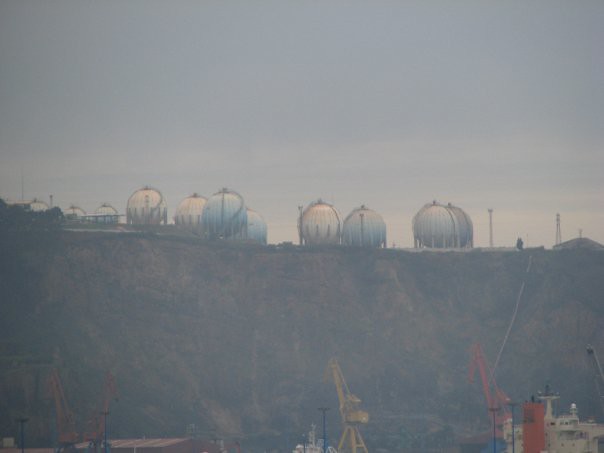This photograph captures a steep, rocky cliff with a construction site nestled at its base. The scene is hazy and slightly blurred, giving it a dull and overcast ambiance. Above the cliff, the sky is a muted blue, streaked with whispering clouds. Dominating the upper part of the cliff are several large, spherical white tanks—possibly for water or fuel—arranged in pairs. These simple, bulbous structures create a stark contrast against the rugged terrain. Below, in the ditch at the bottom of the cliff, various construction equipment is visible, including a prominent yellow crane at the center and a secondary reddish crane to the right. A third, fainter crane can be spotted to the left. Additionally, a power line tower rises in the far right background, and a small building, likely serving as a headquarters, is also discernible on the right. Despite the cloudy and faded quality of the image, the detailed scene conveys an ongoing construction effort in a challenging, mountainous landscape.